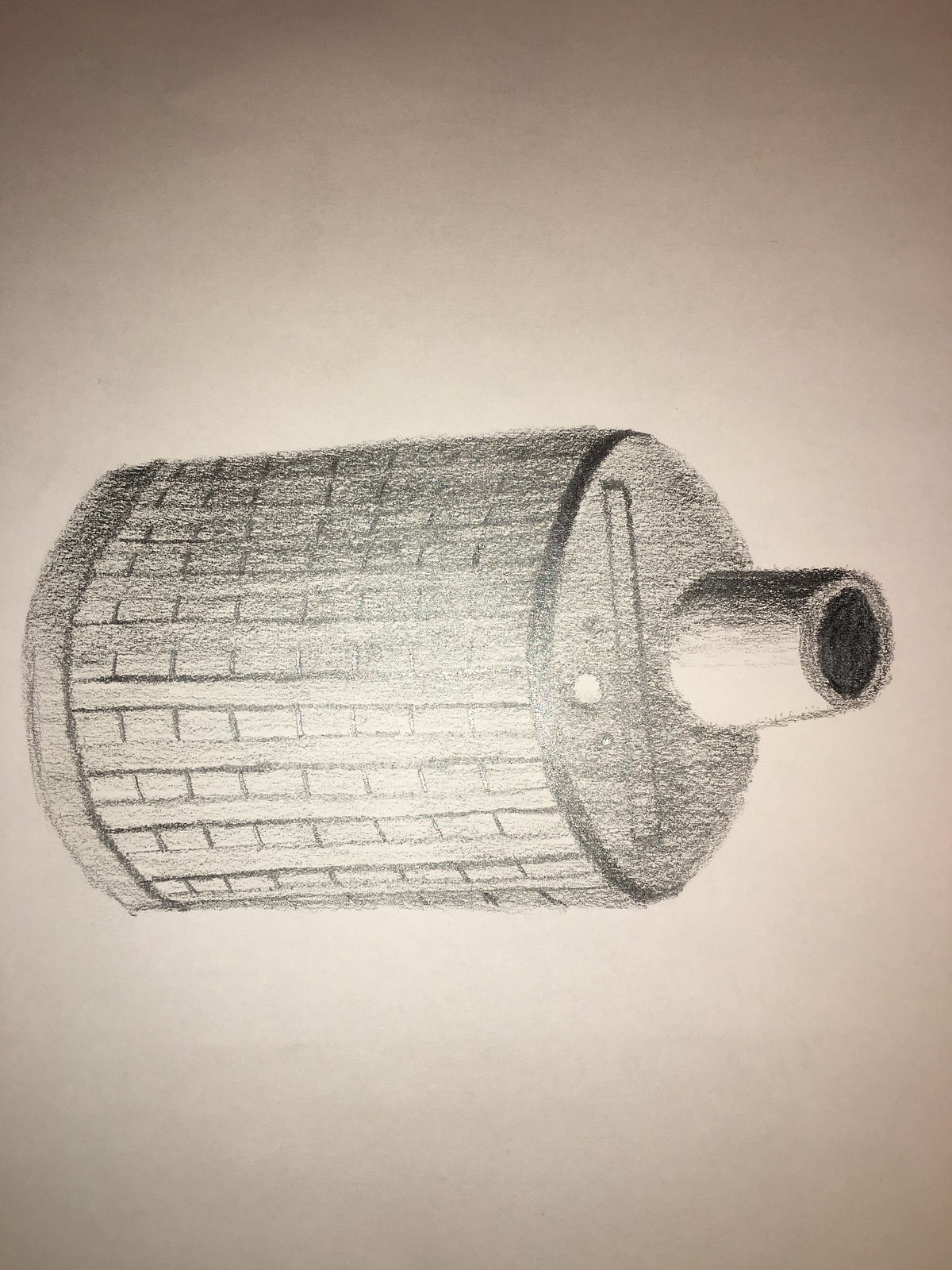The image showcases a highly detailed pencil sketch of a cylindrical object, resembling either an exhaust canister for a car or a barrel-like structure. The object is positioned horizontally across the page, complete with intricate details such as beams running horizontally and vertical lines indicating segmented paneling. On the right side of the cylinder, a semi-cylindrical extension features a prominent black circle signifying an open end. The sketch is monochromatic, rendered meticulously using graphite to create shadows and depth, capturing the object's three-dimensional form. The paper appears to have a subtle gradient from dark to light beige, suggesting it might be a scan or a photo of a page from a sketchbook, possibly by a student or amateur artist. The overall composition hints at the artist's effort to depict the object with considerable attention to detail and shading.